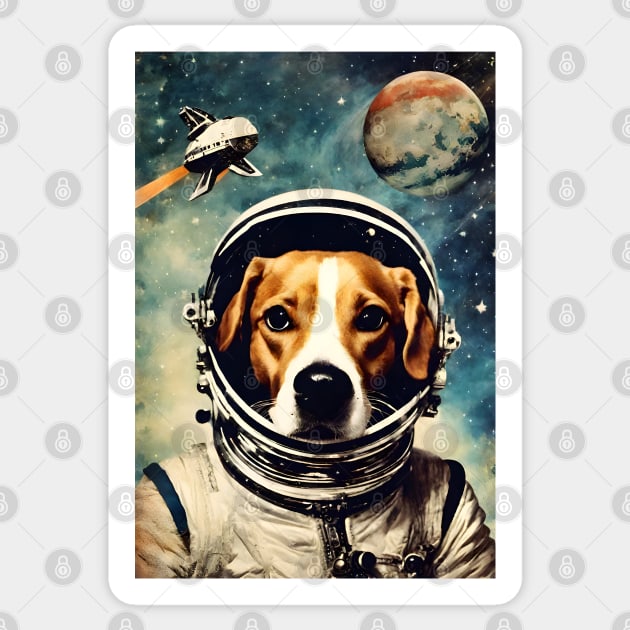This is a detailed digital graphic illustration resembling a portrait, akin to a baseball card. Central to the image is a light to medium brown dog with a black nose, floppy ears, and a white muzzle. The dog is donned in an old-timey astronaut helmet and suit, showcasing the shoulders and upper chest of the ensemble. Set against a backdrop of outer space, the scene features a star-studded dark blue and green swirled sky, a red, white, green, and blue planet, and a white and black spaceship emitting an orange beam in the top left corner. The entire illustration, presented on a gray background with a white border, is overlaid with a repeating watermark depicting a padlock symbol within a circle.